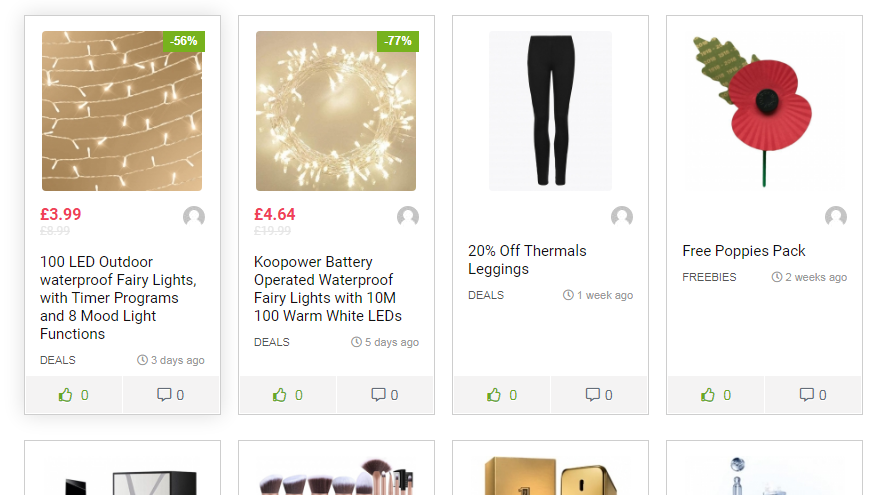The image showcases what appears to be an online shopping site. The layout includes eight thumbnail links arranged in two rows, each containing four items. 

In the top left corner, there is a product listing for "100 LED Outdoor Waterproof Fairy Lights with Timer Programs and Eight Mood Light Functions," priced at £3.99, highlighted in red. The product description and image of the fairy lights are displayed below the title.

To its immediate right, another listing features "COU Power Battery Operated Waterproof Fairy Lights" with 10 meters and 100 warm white LEDs, priced at £4.64. An image of these lights is also included above the product details.

Continuing to the right, there is a listing for black thermal leggings, advertised with a 20% discount. The listing includes an image of a pair of black leggings.

Next to the leggings, there is an item described as a "Free Poppies Pack." The accompanying image, which seems to depict artificial flowers, is not entirely clear about what the product actually is.

The second row of items is partially visible but is cut off, making it impossible to provide further details or descriptions of those products.